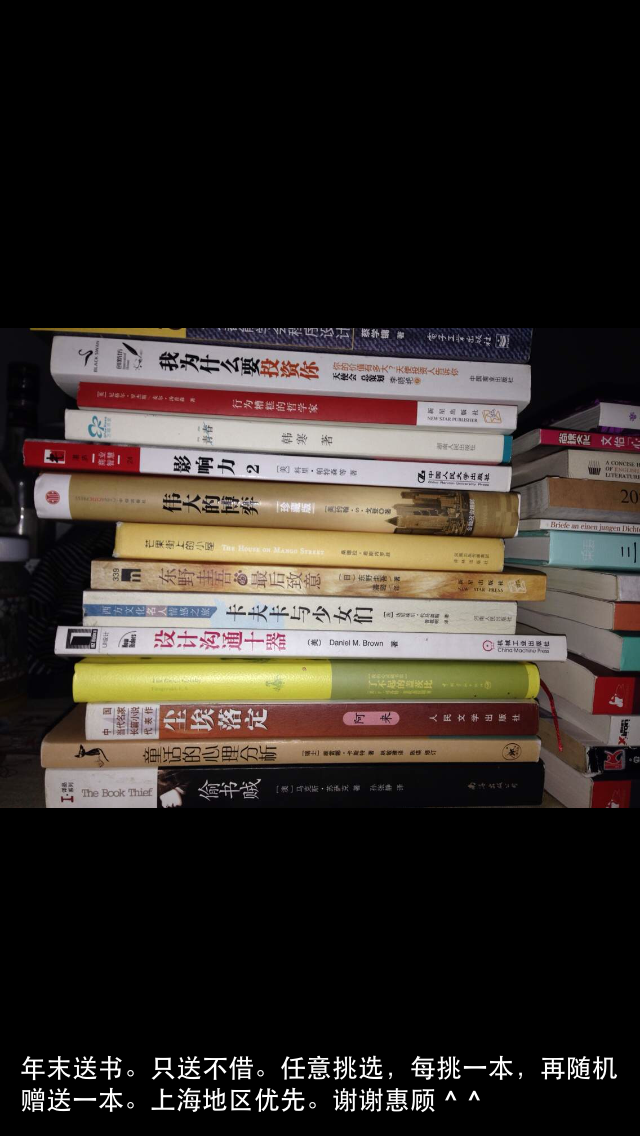The image is a vertically oriented rectangle dominated by a stark black background. The top third of the image and the bottom third are occupied by large, horizontal black rectangles. Between these two black expanses lies the central focus: a nearly square section filled with stacks of books, all laid horizontally and one on top of the other. 

The books exhibit a variety of colors, including red, white, yellow, green, blue, beige, brown, and black. They also display diverse languages on their spines, predominantly composed of Asian characters which are possibly Chinese, Japanese, or Korean. These spines are adorned with text in black, red, blue, and white, but their exact meanings remain unreadable due to the foreign script. 

Among the stack, the books feature a mix of paperbacks and hardcovers. Notably, one book with a beige cover bears an emblem resembling the Japanese flag (a white flag with a red circle). Another book's spine is revealed to have the English title "The Book Thief."

On the bottommost black rectangle, there are additional white characters, also in an Asian language, that add more to the mystery of the text. To the right of the main stack, a second, partially visible stack can be seen, cropping off the image and hinting at more books beyond the frame. The entire scene evokes a sense of scholarly abundance set against a minimalist, almost solemn backdrop.